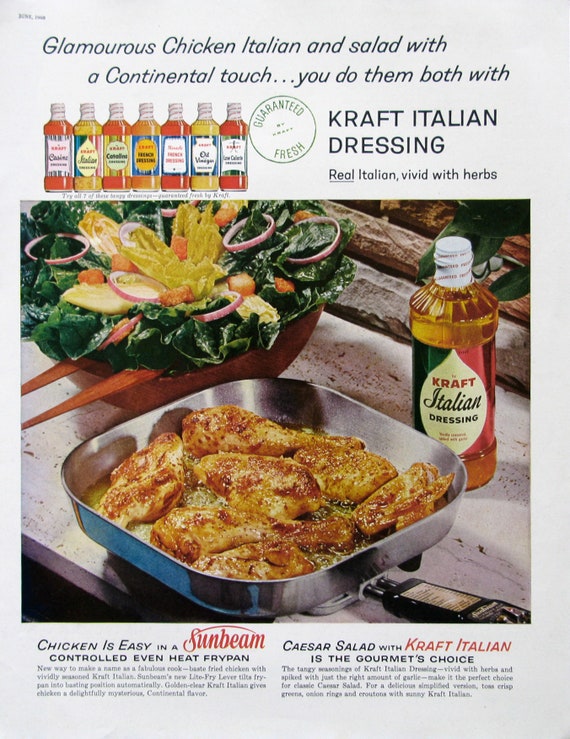This image features a vintage advertisement for Kraft Italian Dressing. At the center of the scanned ad, a large wooden bowl brimming with a vibrant, crafted salad is prominently displayed, accompanied by a square skillet sizzling with glistening pieces of cooked chicken. Positioned beside the skillet is an unopened bottle of Kraft Italian Dressing, adorned with an Italian flag-themed logo. The top of the advertisement reads: "Glamorous Chicken Italian and Salad with a Continental Touch. You do them both with Kraft Italian Dressing. Real Italian, vivid with herbs."

Further emphasizing the product’s versatility, the upper left corner showcases seven different bottles of Kraft dressings under the heading: "Try all seven of these tangy dressings, guaranteed fresh." At the lower section, two captions underscore the dual promotion - one about the ease of cooking chicken "in a Sunbeam controlled even heat frying pan" and the other endorsing "Caesar salad with Kraft Italian as the gourmet's choice." Both captions are followed by detailed descriptive paragraphs in fine print. The overall composition, with its nostalgic photographic style and period-specific elements, reflects a bygone era of culinary advertising.